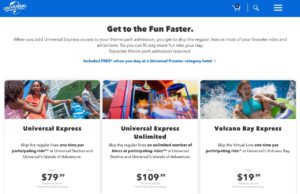The image is a detailed promotional graphic for Universal Studios' various attraction passes. The central focus is on the Universal Studios logo, depicting the iconic globe with the word "Universal" wrapped around it, indicating that this pertains to the renowned Universal Studios theme park.

The image is divided into several sections, each promoting different Universal Express options:

1. **Universal Express - $79.99**: This section shows a happy family walking through what appears to be a lively themed street within the park. Text accompanying the image highlights the cost and benefits of the Universal Express pass, allowing guests to enjoy attractions with reduced wait times.

2. **Universal Express Unlimited - $109.99**: The middle section, showcasing another cheerful family, possibly entering a restaurant, emphasizes the unlimited aspect of this pass, offering even more convenience and access throughout the park.

3. **Volcano Bay Express - $19.99**: The final section features a woman joyfully riding a raft down a thrilling water slide, promoting the express pass for Volcano Bay, Universal's water theme park. This pass provides reduced wait times for specified water attractions.

The background of the graphic is predominantly white with blue banners at the top, contributing to a clean, professional look. Additional features include a search icon (magnifying glass), a shopping cart icon for easy purchases, and a hamburger menu icon for expanded navigation options. The clean layout and vivid imagery successfully convey the excitement and benefits of Universal Studios' express passes.